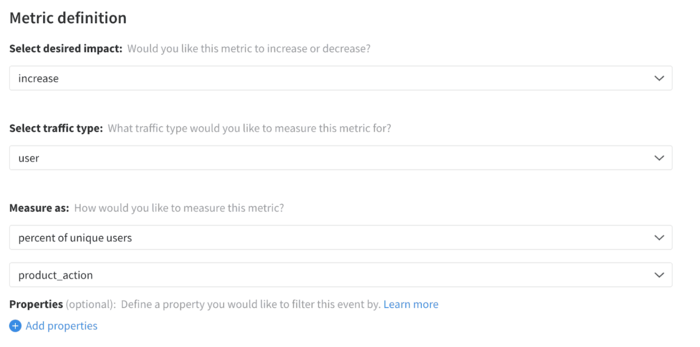The screenshot is set against a solid white background, and features a detailed metric configuration interface. In the upper left corner, bold black text reads "Metric Definition." Directly beneath, smaller black text states "Select desired impact," accompanied by a gray-text prompt to the right asking, "Would you like this metric to increase or decrease?" A dropdown box below this displays the word "Increase," indicating the selected option. 

Further down, another bold black text heading reads "Select Traffic Types," with the accompanying gray text question, "What traffic type would you like to measure this metric for?" The dropdown box below this contains the word "User."

Next, the section labeled "Measure As" poses the question, "How would you like to measure this metric?" in black text, with the dropdown box containing the phrase "Percent of unique users" in gray text.

The following white box is labeled with "Product" and "Product Action" in gray text, accompanied by another pull-down option. At the bottom, bold black text titled "Properties" asks you to "Define a property you would like to filter this event by."